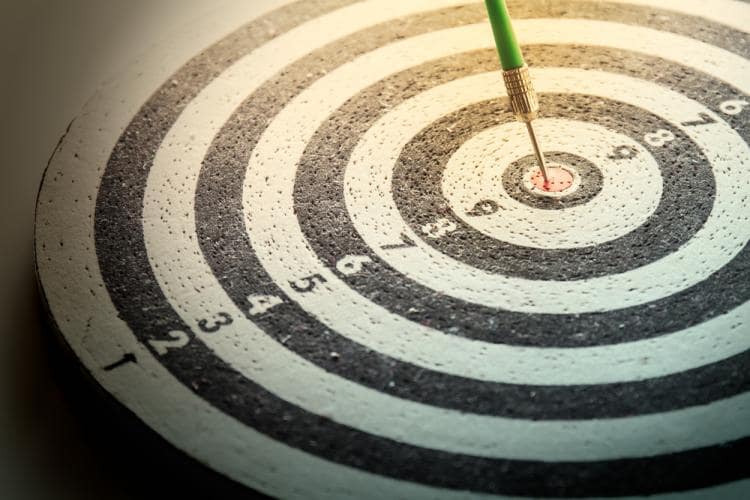The image depicts a well-used dartboard laying flat on a white surface, with around 75% of its circumference visible. The dartboard features concentric black and white rings, alternating in color, with black numbers on the white rings and white numbers on the black rings. These numbers range from 1 at the outermost ring to 9 near the center. At the heart of the dartboard is a red bullseye, into which a green dart with a silver tip is firmly lodged, indicating a perfect shot. The used condition of the dartboard is evident from numerous holes, predominantly concentrated on the left side. The dartboard consumes most of the frame, with only a small section of the table surface visible around it.